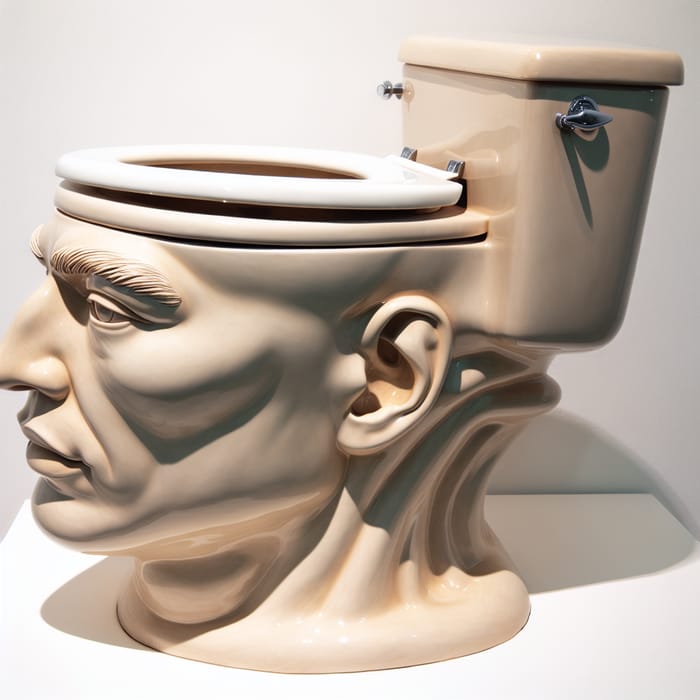The image captures an exceptionally unique and surreal toilet, primarily serving as an ornate sculpture of a man's head. The head features high cheekbones, a profound Roman-style nose, a strong chin, and thick, very detailed eyebrows. The sculpture is crafted in natural, muted clay-colored tones, giving an earthy, off-white appearance. The toilet seat, however, is a standard white seat positioned at the top of the man's head. The flush mechanism and hardware, including silver handles, are typical and attached to a light tan-colored water tank. The man's face is oriented westward, away from the back of the toilet where the tank is attached. Despite its sophisticated artistic elements, the toilet appears functional but could also serve solely as a piece of art. The background of the image is a simple whitish setting, and the toilet rests on a white floor, emphasizing its detailed craftsmanship and creative design.